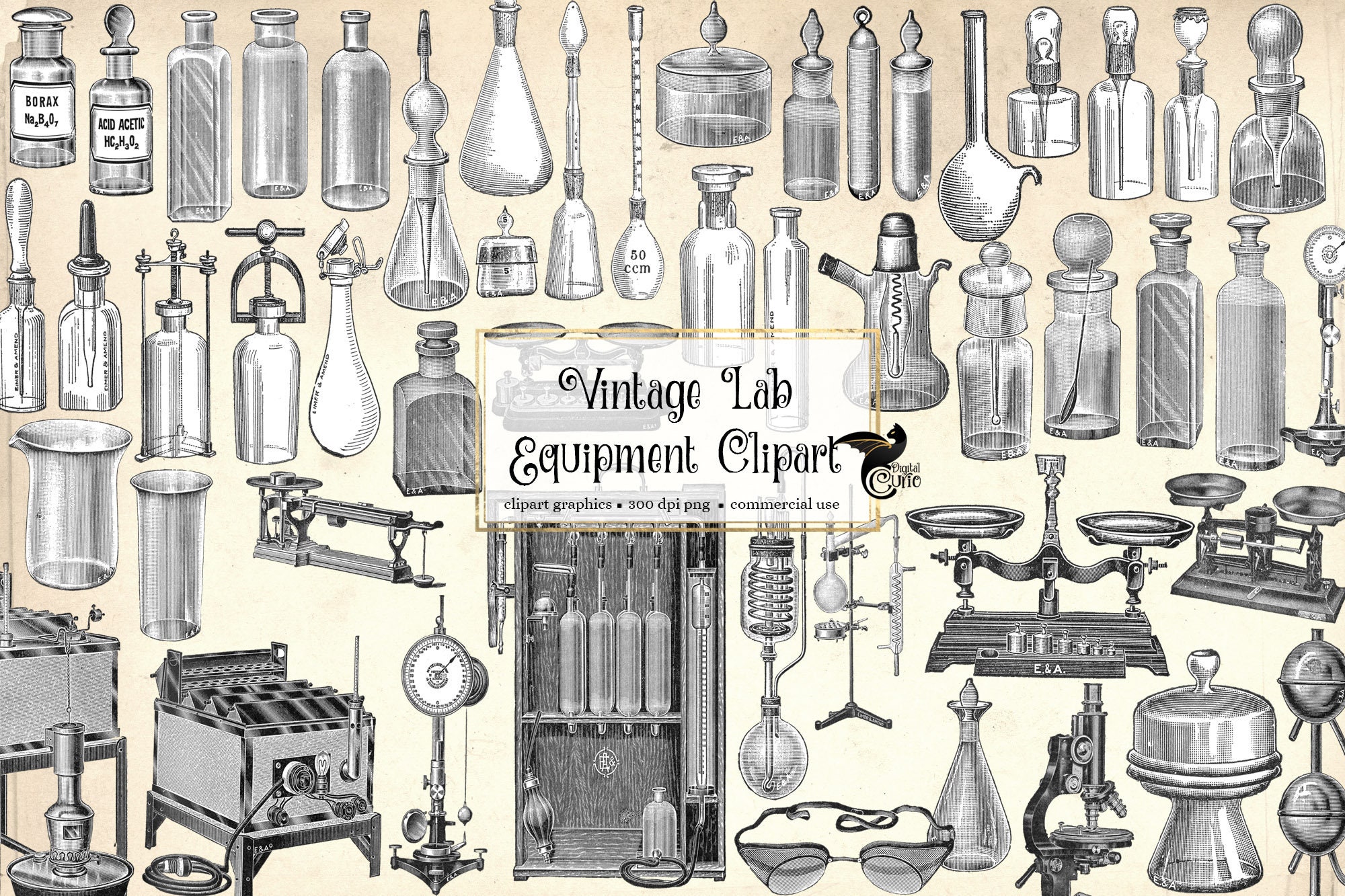This image features a meticulously hand-drawn black and white diagram showcasing various vintage laboratory equipment, skillfully illustrated for clip art purposes suitable for commercial use. The diagram is designed at a high resolution of 300 dpi. At the center of the image is a transparent white rectangle bearing the title "Vintage Lab Equipment Clipart" in black text. Surrounding this central title is a yellow frame, set against a textured yellowish background.

The detailed illustrations include a diverse array of classic lab instruments, such as glass jar bottles, beakers, flasks, burners, traditional scales, and microscopes—meticulously sketched to highlight their 3D dimensions. Various types of glassware are prominently featured, displaying over 50 different variations of these old-school experiment tools. Additionally, items like goggles and other essential laboratory apparatus are thoughtfully rendered, reflecting their historical significance. The entire collection is drawn in pencil, emphasizing the intricate detail and craftsmanship of each piece.